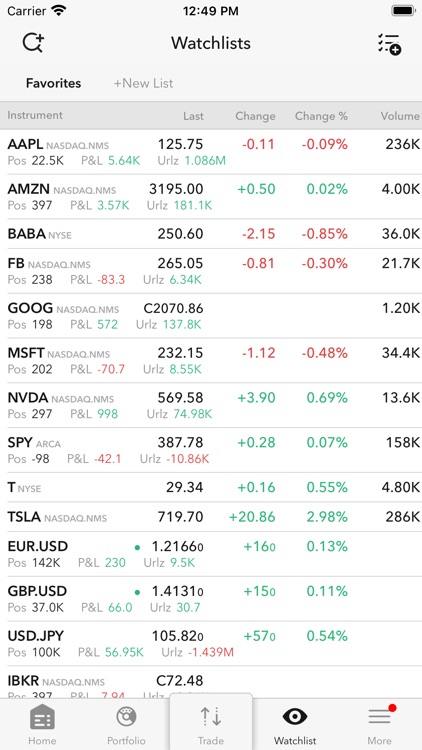This is an image of a stock trading website displayed on a smartphone. The phone's status bar shows that the carrier is named "Carrier," with a strong signal connection, and it is 12:49 PM. The battery icon indicates a full charge. 

The website is organized into several sections. At the top, there is a plus sign above three vertical lines, accompanied by check marks on the left side. Below, a "Favorites" section appears with a gray circle on the right side above it, and a "Plus New List" option in light gray next to it.

The main section lists various stocks under different categories: "Instrument" for the stock symbols, "Last" for the latest stock price, "Change" for the daily price change (with green pluses representing gains and red negatives representing losses), "Change %" for the percentage change (also color-coded in green for ups and red for downs), and "Volume" for the trading volume, where "K" denotes thousands.

At the bottom, partially cut off, is a navigation bar in gray. It includes:
- "Home" in black text,
- "Portfolio," represented by a round black and white icon,
- "Trade," signified by arrows pointing up and down,
- "Watchlist," indicated by a black eye icon,
- "More," symbolized by three horizontal lines with a red dot on the top line and "More" text underneath.

The overall interface suggests a comprehensive, user-friendly experience for tracking and managing stock investments.